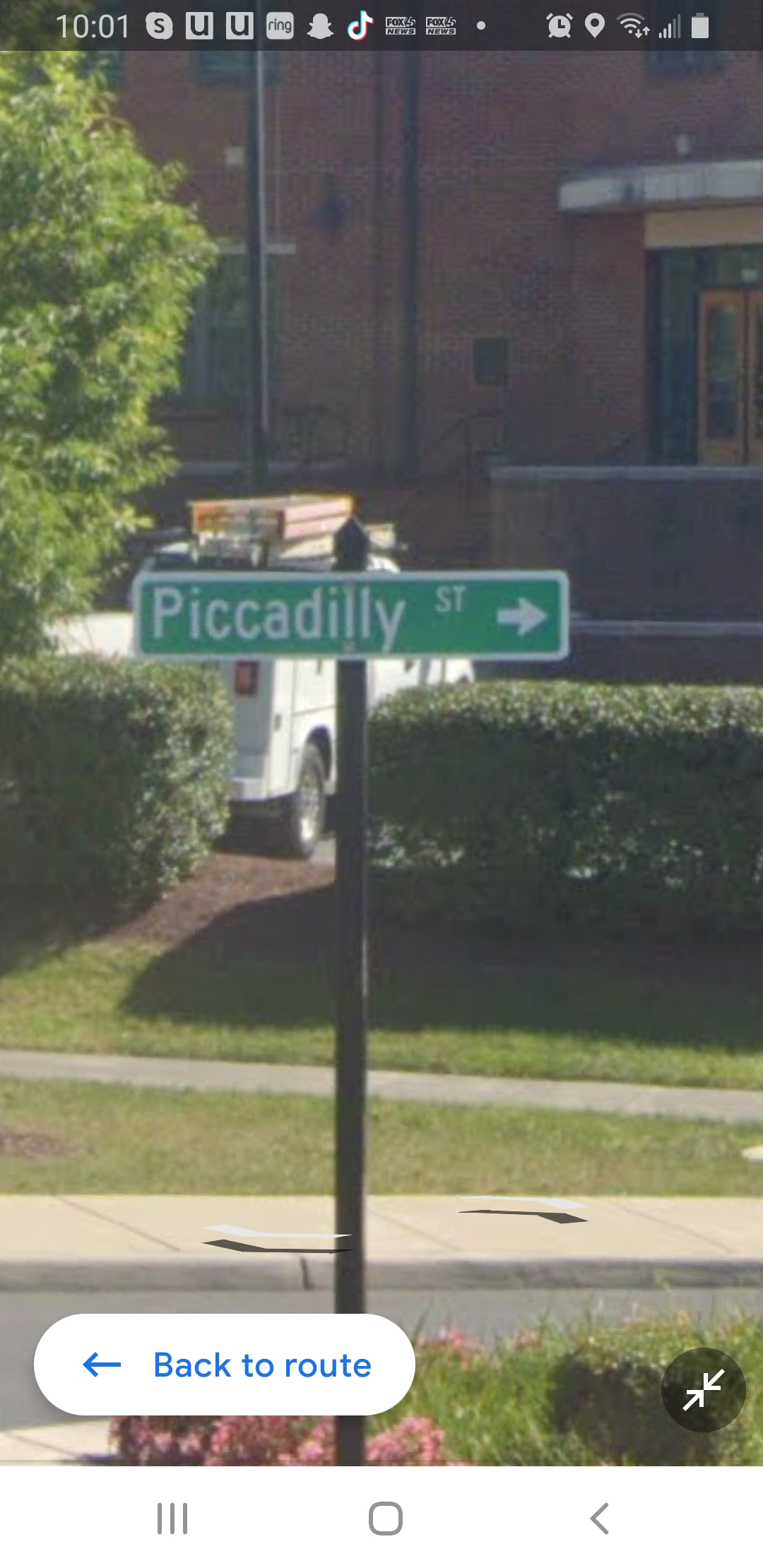The image appears to be a screenshot taken from a phone, possibly from a Street View on RoboMaps. At the very top, the phone's notification bar displays a time of 10:01, along with various app icons including Skype, UltiPro, Ring, Snapchat, and TikTok, and indicates that the battery is mostly full. The focal point of the image is a rectangular road sign with a white outline and a green center that states "Piccadilly Street" with a white arrow pointing to the right. This sign is mounted on a black pole surrounded by green grass and pink flowers at its base. In the background, there is a gray building with brick walls, a tree on the left, and two neatly trimmed green hedges in the middle. A white truck with an orange ladder on it is also visible. Additionally, there are circular signs—a blue one with an arrow pointing left that says "Back to Root," and a light gray one with two white arrows pointing at each other. The image includes the edge of a road and two sidewalks. A black banner at the top reads "1001" followed by a dollar sign and other unidentifiable symbols.